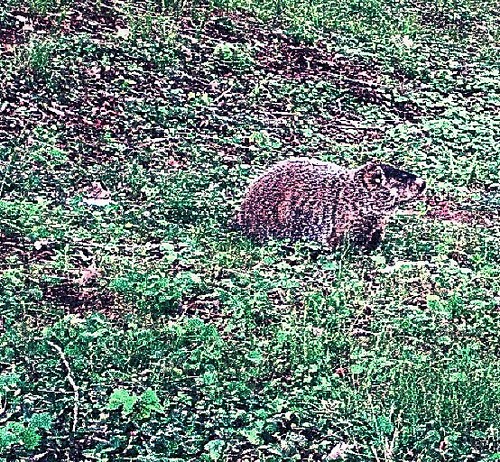The image captures a small badger standing in the midst of a green field, almost blending seamlessly into its surroundings. The field is dotted with small grasses, mint plants, weeds, and twigs, giving it a somewhat sparse yet lively appearance. The badger is positioned in the center-right of the square photo, with its head directed upwards and to the right. The badger's fur is an intricate mix of tan, brown, and black specklings, providing effective camouflage against the grassy backdrop. The badger's black nose and darker head, contrasted with its tan-speckled body, make it challenging yet possible to distinguish it from the similarly colored vegetation. The image quality appears grainy, featuring high contrast with numerous white dots scattered throughout, enhancing its textured appearance. The overall scene is tranquil with a rich blend of green foliage and patches of brown dirt and leaves, contributing to an earthy, natural setting.